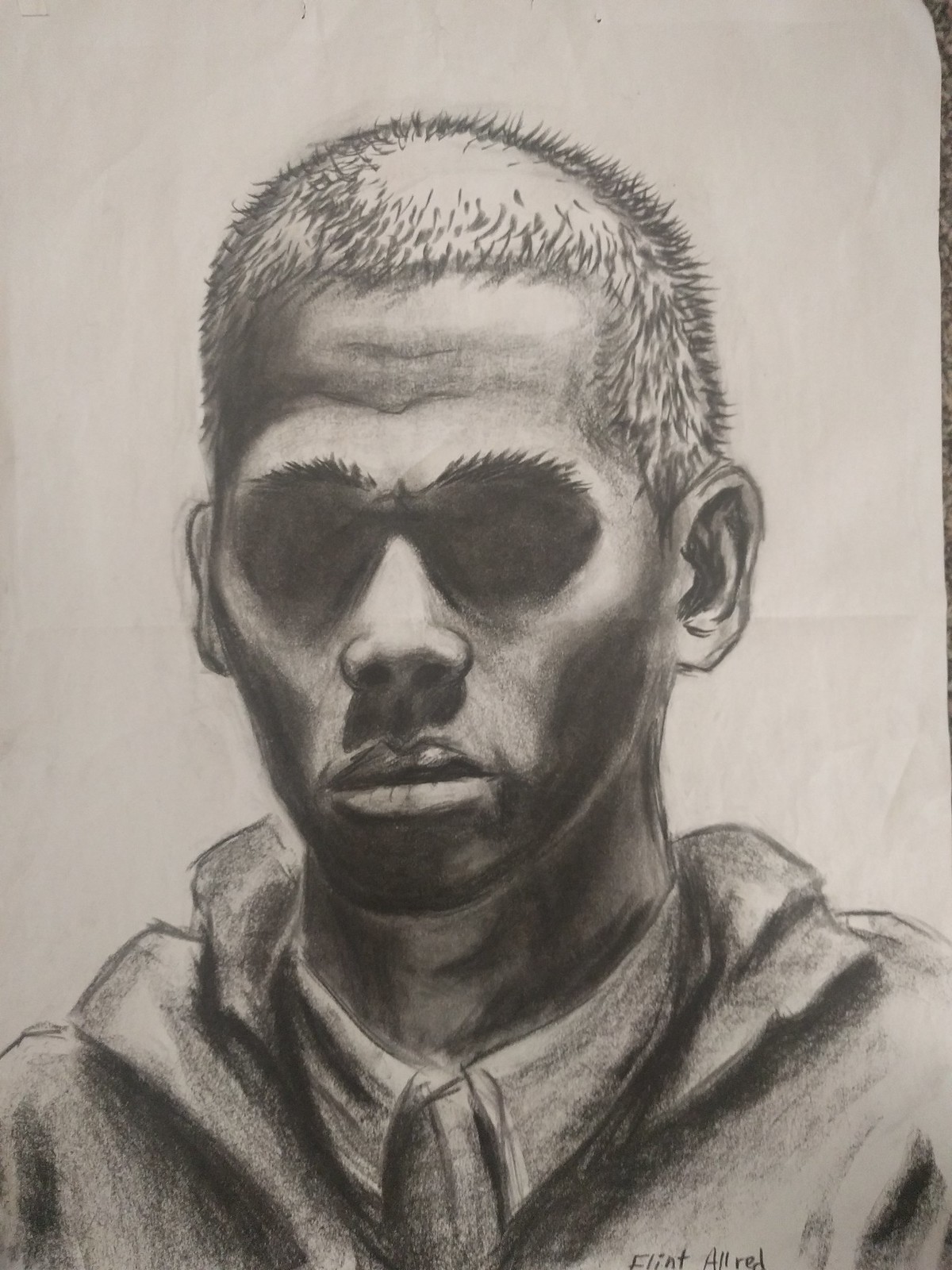This pencil drawing depicts a male figure characterized by short, spiky hair and prominent, bushy eyebrows. The artist has used extensive shading, creating a black-and-white composition with deep shadows that obscure the man's eyes and add depth to his jawline, chin, and neck. The gentleman is dressed in a button-up shirt, layered with a hoodie or a jacket featuring multiple collars, giving his attire a slightly baggy appearance. The artist's signature, "Flint Allred," is visible at the bottom of the drawing, although it is partially cut off.